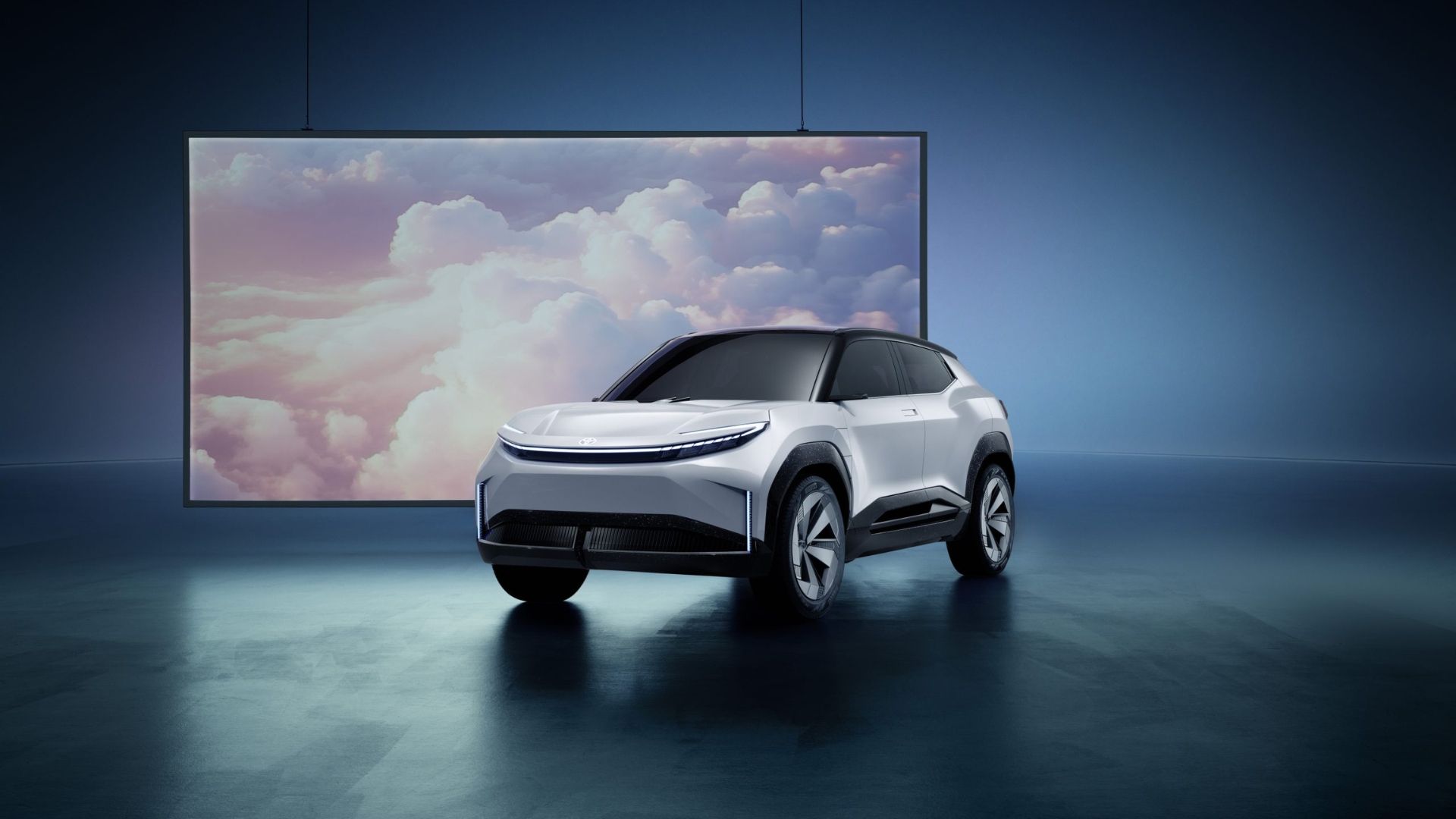The detailed caption for the image, incorporating elements from each description, is as follows:

The image depicts a sleek concept car, an SUV with a modern, futuristic design. The vehicle is primarily gray, with gray rims and black tires, complemented by a black roof and black side panels around the windshield. The standout feature of the car is its single, continuous strip of headlights running across the front. It sits on a highly polished concrete floor, marked with various scuffs and signs of wear, which reflects the car's image subtly. 

In the background, a solid light blue wall provides a cool backdrop to the scene. Suspended from the ceiling by two long, noticeable wires is a large rectangular screen that captures attention with its picturesque display of a cloudy sky. The screen, bordered with a thick black edge, shows a vibrant expanse of fluffy white clouds against a backdrop of orange and blue hues, contributing to a serene and artistic atmosphere. The intentional play between the car's sleek, monochromatic palette and the lively, colorful display behind it creates a compelling visual contrast.